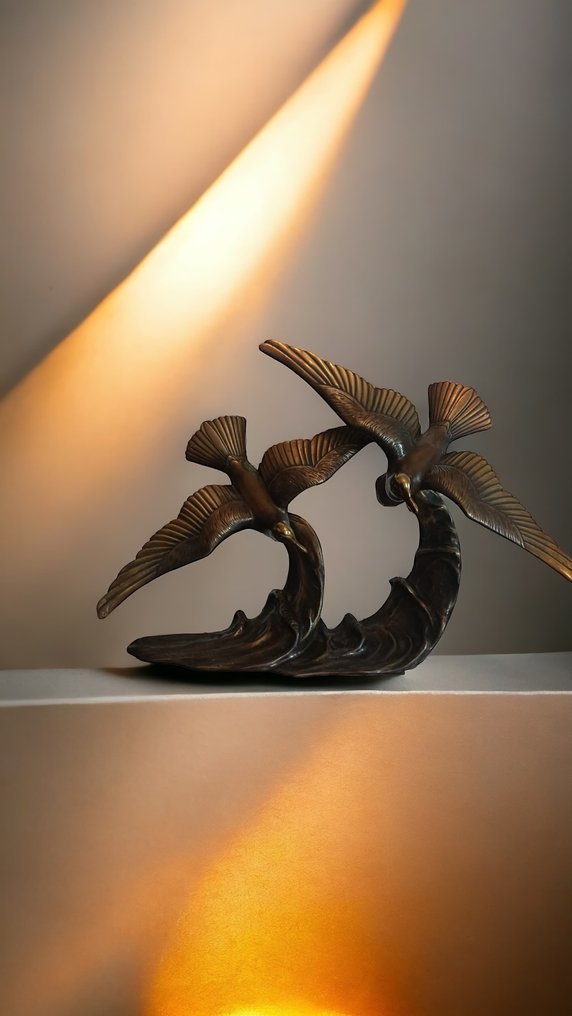The photograph showcases a meticulously crafted, bronze-colored sculpture of two birds diving toward each other against a detailed backdrop that suggests waves. These intricately carved birds, possibly ducks, have outstretched wings featuring detailed designs and finely sculpted tail feathers, indicating the artisan's thorough and skilled craftsmanship. The sculpture is placed on an off-white ledge, occupying the bottom third of the image. The middle third highlights the dynamic forms of the birds and waves, set against a beige wall. Bright, golden sunlight streams in from the top of the image, enhancing the fluid and elegant appearance of the art piece, giving the impression that it is illuminated by sunlight coming through a window.